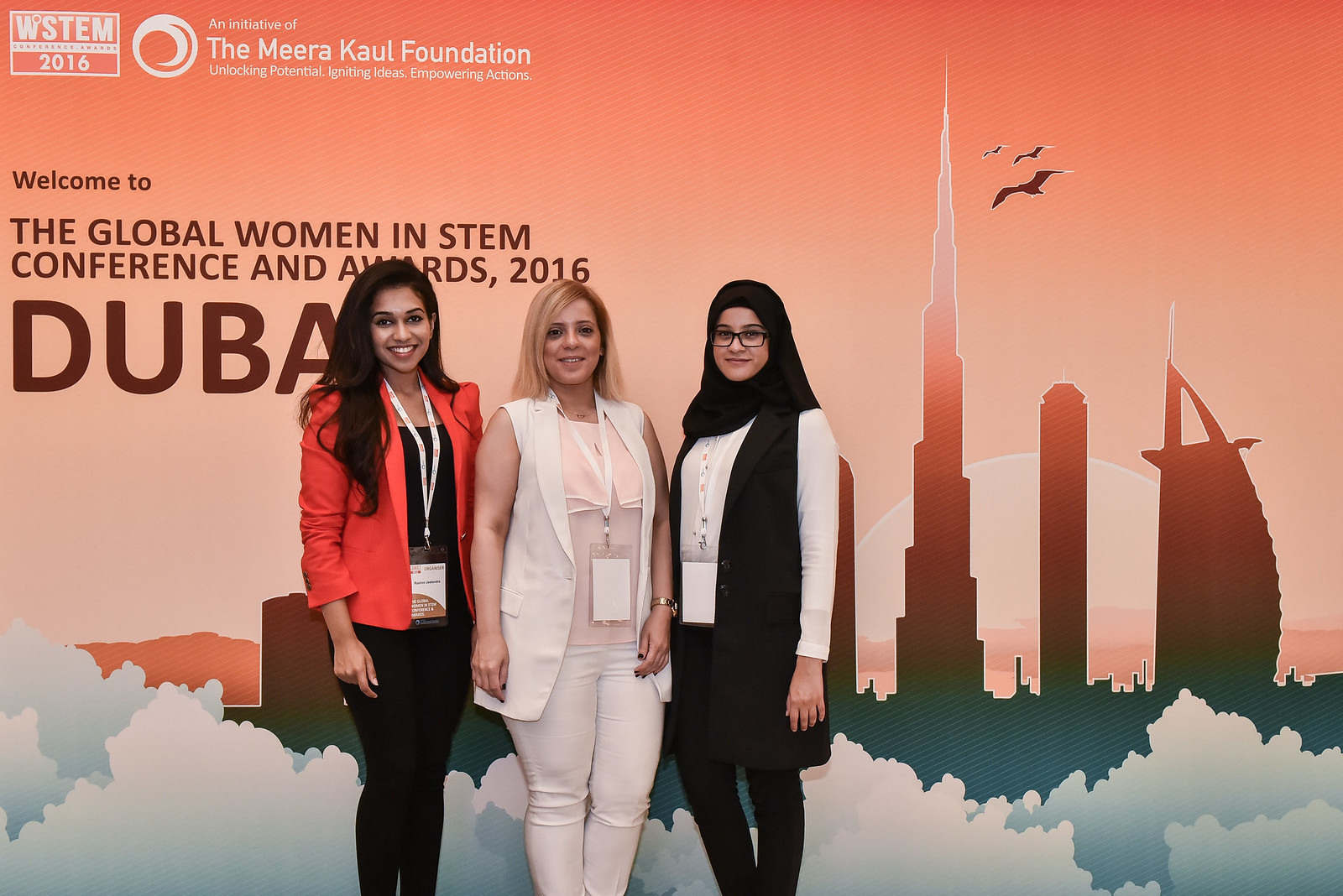This full-color photograph captures three women standing against a backdrop reminiscent of a sunrise, with an orange-to-peach gradient sky and silhouetted buildings beneath a yellowish sun. The scene features dramatic clouds and soaring birds, adding a dynamic visual element. At the top left corner of the backdrop, inside a box, it reads "WSTEM," followed by an unreadable line, and at the bottom of the box, it says "2016." To the right, a logo is accompanied by "an initiative of" in small white print, followed by the larger text "MEERA KAUL Foundation." Below, it states "Unlocking Potential, Igniting Ideas, Empowering Action."

Centrally located, in brown text, are the words, "Welcome to the Global Women in STEM Conference and Awards 2016," with "Dubai" in large brown print beneath it. The women share a focal point in the photograph: 

- On the left, a woman with long black hair dons a red blazer over a black top and black pants, and wears a lanyard around her neck.
- In the middle stands a blonde-haired woman in a sleeveless white vest over a pink blouse and matching pink pants, also with a lanyard.
- The woman on the right wears a hijab, black-frame glasses, a white long-sleeve top, and black pants, complemented by a black vest.

This image radiates a sense of unity and professional accomplishment, underscored by the vibrant cityscape of Dubai in the background, celebrating the Global Women in STEM Conference and Awards 2016.